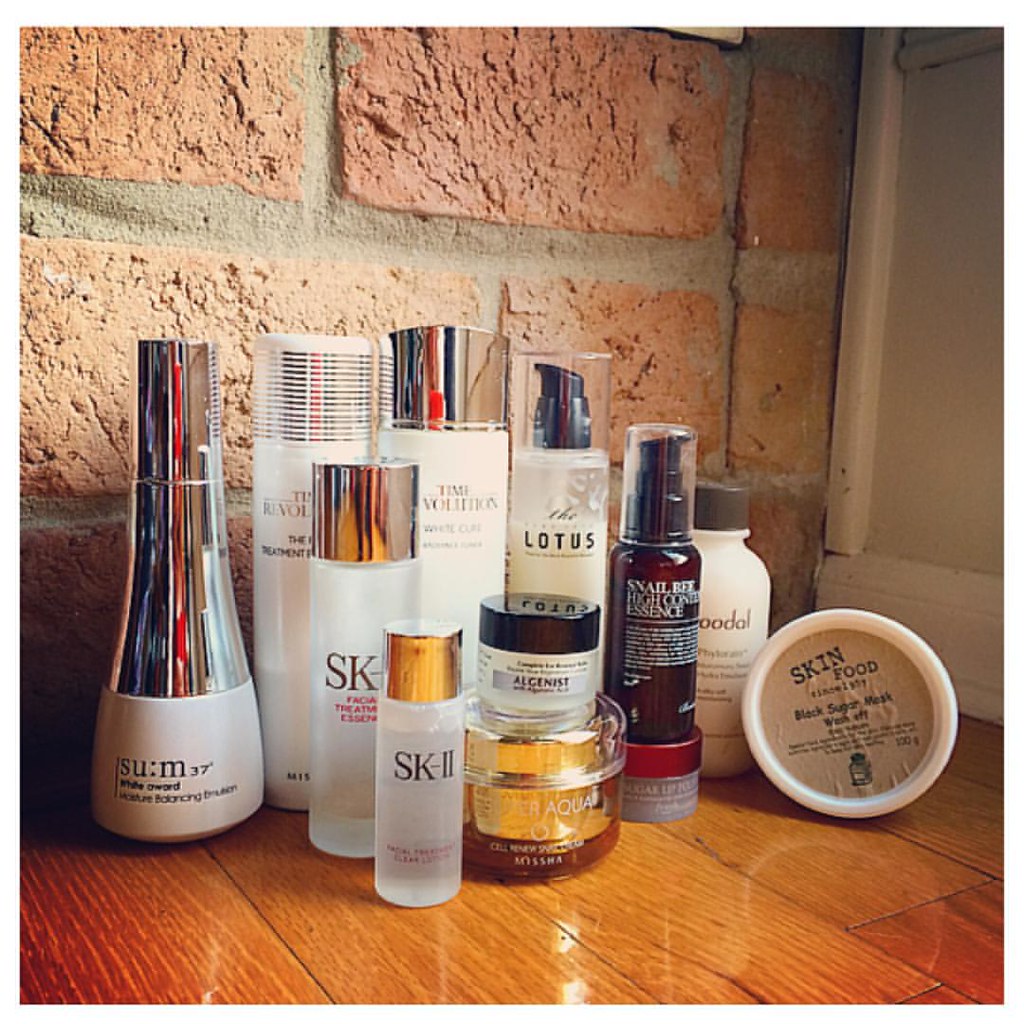The photograph captures an assortment of skincare products meticulously arranged on a glistening hardwood floor. Sunlight streams in from a window, casting a warm glow that highlights the sleek finish of the floor. The products are set against a rustic brick wall, adjacent to which is a white baseboard molding adding a touch of contrast. The collection includes an array of bottles and jars from various brands. Prominently featured are several products from SK-II, including a facial treatment. There are also items from Skin Food, including a Black Sugar Mask Wash Off. Another notable brand is Lotus, with multiple bottles bearing its name. Additionally, there are products from Time Revolution, and a distinctive brown bottle labeled with something that includes "snail" and "essence," intriguingly placed atop a container of sugar lip scrub. The composition exudes a scene of serene morning light illuminating a curated skincare regimen.